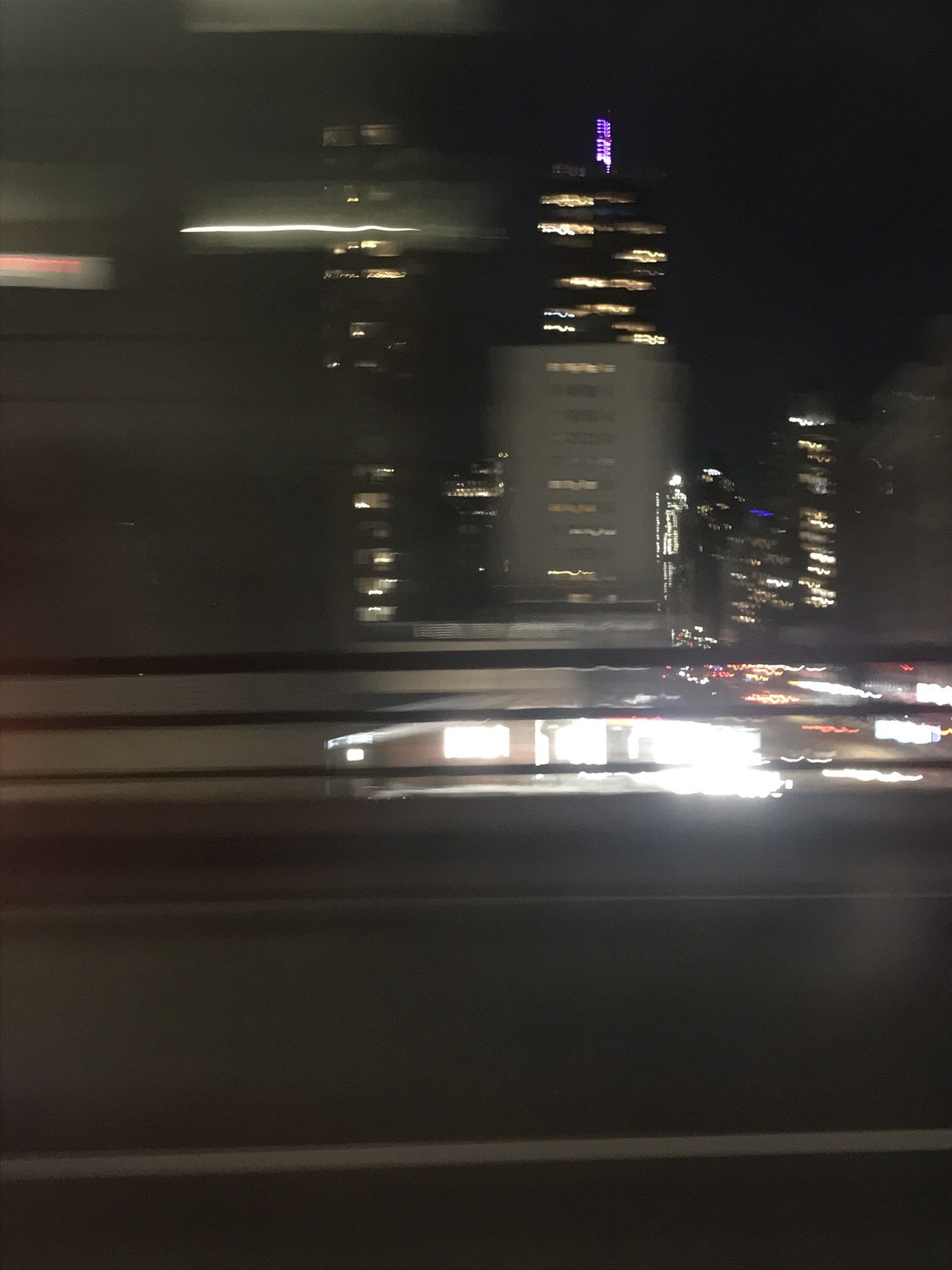In this vertically-oriented, rectangular photograph, we observe a nighttime cityscape captured from the side of a bustling interstate. The image is noticeably blurred, imparting a sense of motion and dynamism. Running through the scene are clear white lines and a gray divider, indicative of road markings common to busy highways. The backdrop is dominated by a series of tall buildings, their illuminated windows forming a striking contrast against the deep black sky. A particularly prominent high-rise stands centrally within the frame, characterized by a white base that evokes the iconic arrangement of the twin towers. Approximately half of the windows across these towering structures emit a warm, glowing light, while streaks of moving lights add an ethereal quality to the photograph, hinting at the ceaseless activity within this urban environment.